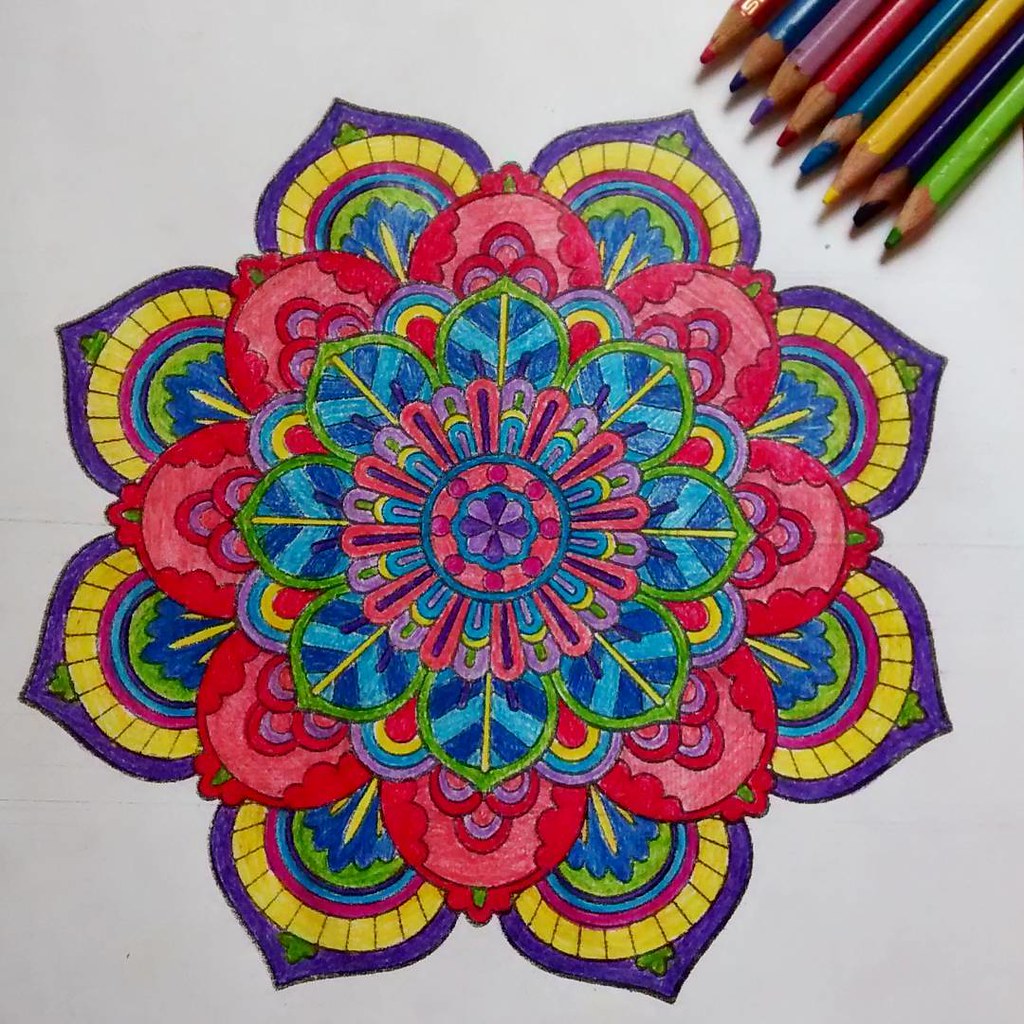This photograph features a detailed color pencil drawing on a white sheet of paper. Positioned in the top right corner are the colored pencils used for the artwork; these pencils include red, dark blue, pink, purple, blue, yellow, dark purple, and green. The central focus of the image is an elaborate abstract shape resembling a lotus flower, showcasing multiple layers of petal-like forms. Each layer alternates in color, creating a vivid, kaleidoscopic effect. Starting from the pink-centered core, blue flowers surround it, followed by layers featuring pink, yellow, purple, and blue petals. The overall design exudes a zen-like quality, akin to adult coloring books or intricate mandala patterns, with the petals' colors transitioning through various shades of blue, red, green, and purple, giving it a harmonious and mesmerizing appearance.